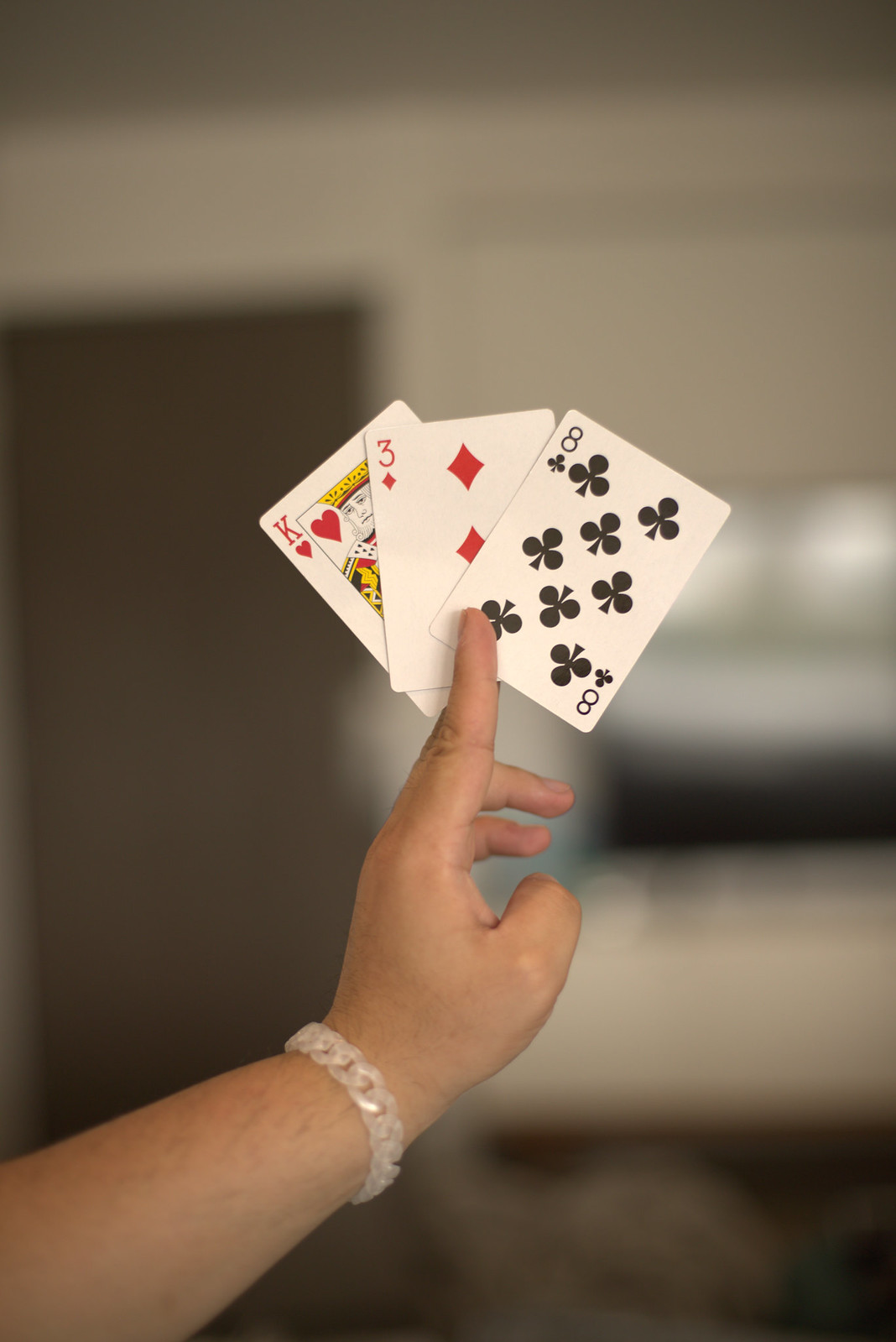This photograph captures a first-person perspective of an individual holding three playing cards in their left hand. Their index finger is extended outward, while the ring finger and pinky are bent inward, and their thumb is slightly crooked. The person is wearing a white plastic bracelet on their wrist, and some hair is visible on their arm. The three cards include the King of Hearts, the Three of Diamonds, and the Eight of Spades. 

The background is softly blurred, suggesting focus on the cards and hand. The room is well-lit with white walls and features a dark wood door to the left. The floor appears to be dark-colored as well. Centrally located is a large piece of white furniture with a black square centerpiece and some lighting fixtures toward the top. The overall ambiance suggests a clean and minimalist interior design.